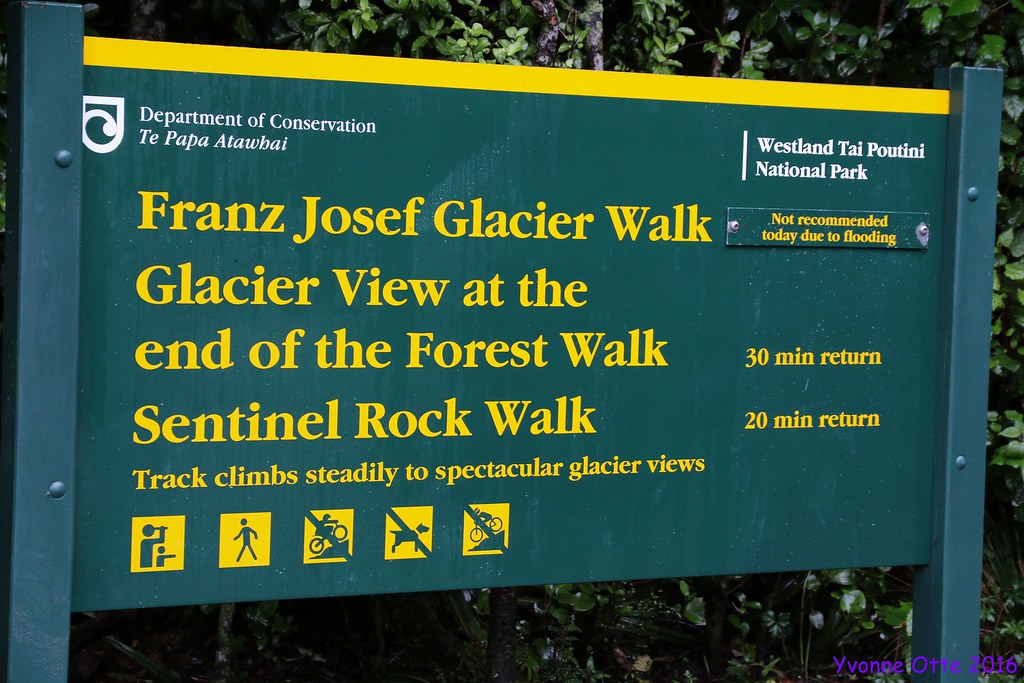This detailed photograph captures a prominent green signpost located in Westland Tai Poutini National Park, surrounded by a backdrop of lush greenery and trees. The sign, supported by posts on either side, features a yellow border at the top and contains comprehensive information in yellow text. In the upper section, the left side reads "Department of Conservation Te Papa Atawhai," accompanied by a two-dimensional emblem, while the right side displays the park's name.

At the center of the sign, bold yellow letters announce "Franz Josef Glacier Walk." Directly beneath, it states "Not recommended today due to flooding." Further down, the sign outlines two walking tracks: "Glacier View at the end of the forest walk, 30-minute return," and "Sentinel Rock Walk, 20-minute return. Track climbs steadily to spectacular glacier views." 

The lower portion of the sign features five small square icons. These icons depict: two people sightseeing, a person walking, a cyclist with a slash through it indicating cycling is prohibited, a dog with a slash through it showing dogs are not allowed, and a downhill bicycle with a slash through it, again indicating prohibition. The vivid details of this sign provide clear guidance and restrictions for park visitors.